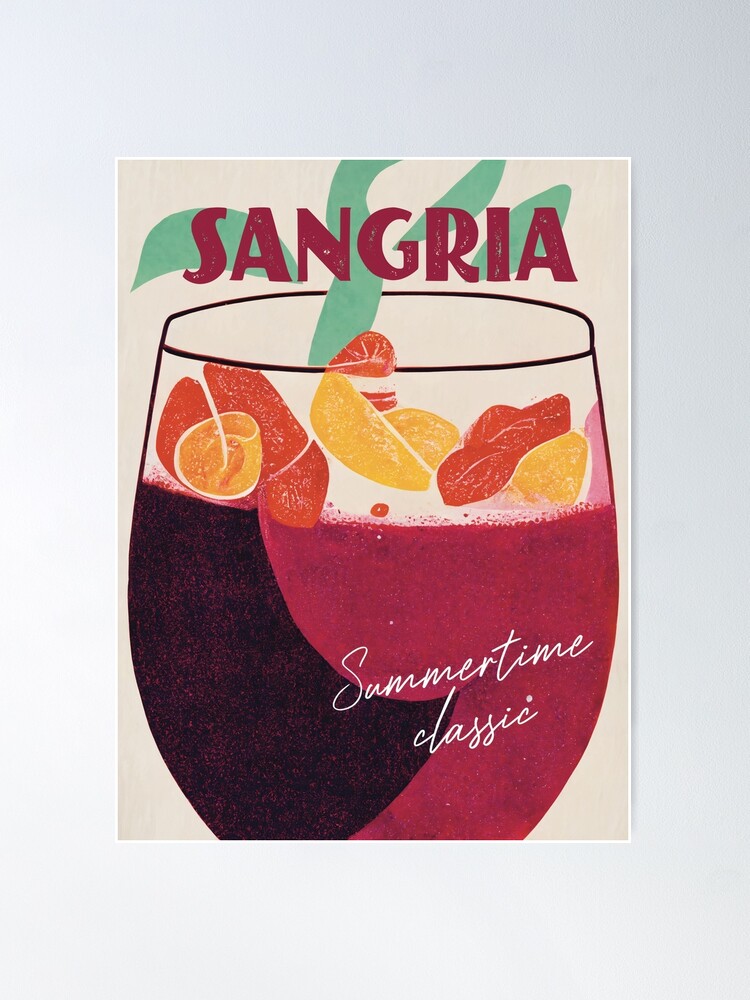The image is an illustrative poster for a sangria advertisement, set against a grey background with a thin white frame. Dominating the composition is a large glass of red sangria, which appears 75% full. The sangria is a rich maroon color on the right side, blending into a darker, blackish hue on the left. Floating atop the drink are slices of orange and yellow citrus fruits, accentuating the summery theme. Green garnish adds a fresh touch and weaves through part of the bold red bubble letters spelling "SANGRIA" across the top. Below, in elegant white italic script, the words "Summertime Classic" are inscribed, reinforcing the seasonal appeal of the beverage. The overall palette consists of inviting red, maroon, orange, yellow, and green tones, all outlined in black.